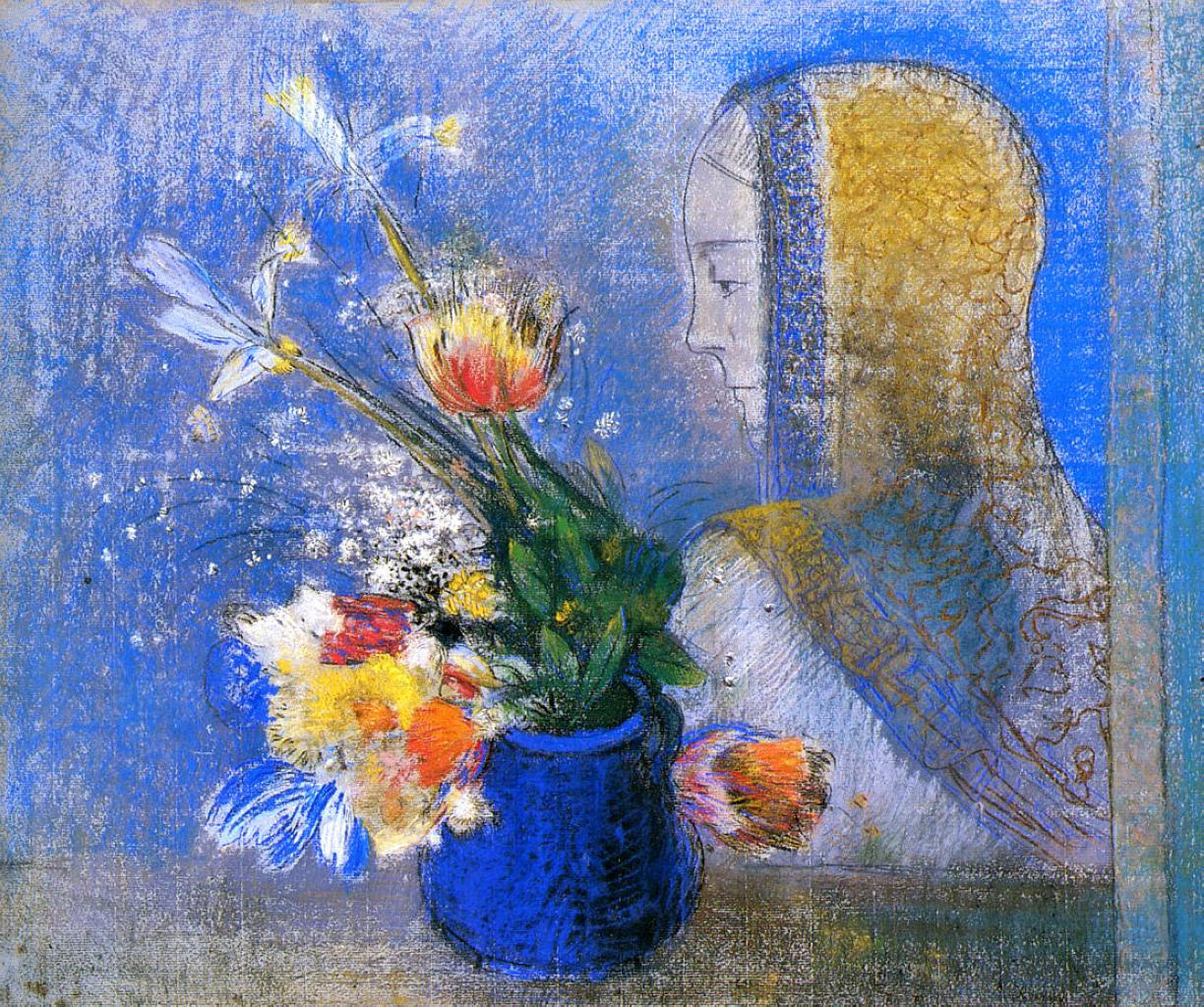This detailed and descriptive caption for the painting synthesizes the information from the three provided voice captions:

"Odilon Redon's 'Meditation' is a captivating color pastel drawing in landscape orientation, characterized by the texture of chalk. The painting features a round, medium blue vase adorned with various vibrant flowers, including a blue iris angling towards the upper left, sprays of white blossoms, and several orange and yellow flowers, with a notable central blossom resembling a yellow and red tulip. Green leaves accentuate the floral arrangement, which is set against a tan windowsill. To the right, a woman is depicted in profile, her gaze directed slightly downward, suggesting a meditative state. She wears a shawl with a gold design and blue border that covers her head and drapes over her shoulders, with her expression and face rendered in black and white, devoid of color. Below the shawl, a glimpse of a white dress is visible. The background is beautifully interwoven with shades of blue and white, evoking a serene and contemplative atmosphere. The painting belongs to the Symbolism movement and reflects the Impressionist style's influence, highlighting emotional depth and the subtle interplay of colors and forms."